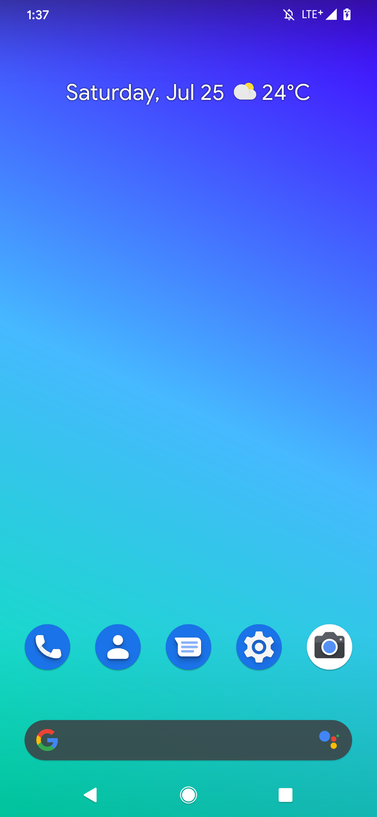This is a detailed caption for the given description of a screenshot:

---

This screenshot, taken from a smartphone, displays a minimalistic vertical layout typical of a mobile device's home screen. At the top of the screen, the status bar is visible, showing the time as 1:37 in the upper left corner. The upper right corner features several icons: a bell symbol with a line through it indicating that notifications are silenced, the text "LTE+" indicating the network connection, a white triangle symbol, and a battery icon showing the current battery status.

Centrally, the upper portion of the screen provides the date and weather details in white text. The date is "Saturday, July 25," followed by an icon of a cloud with a small sun, and a temperature indication of "24 degrees Celsius."

The background of the screen features a gradient color scheme, transitioning from blue at the top to a greenish tone towards the bottom, creating a smooth ombre effect.

Positioned near the bottom of the screen are five circular icons with blue backgrounds and white symbols. From left to right, these icons include:
1. A white telephone icon,
2. A white person silhouette,
3. A white document symbol with text lines,
4. A bolt symbol,
5. On the far right, a white circle with a black camera icon that has a blue lens.

Just above these icons is a prominent black Google search bar, which is horizontally oval-shaped with a distinct "G" for Google on the left side.

At the very bottom of the screenshot, the standard navigation icons are present, consisting of a white triangle, a white circle, and a white square aligned from left to right.

---

This detailed caption provides a clear and thorough depiction of the image, highlighting all visual elements and their arrangement.